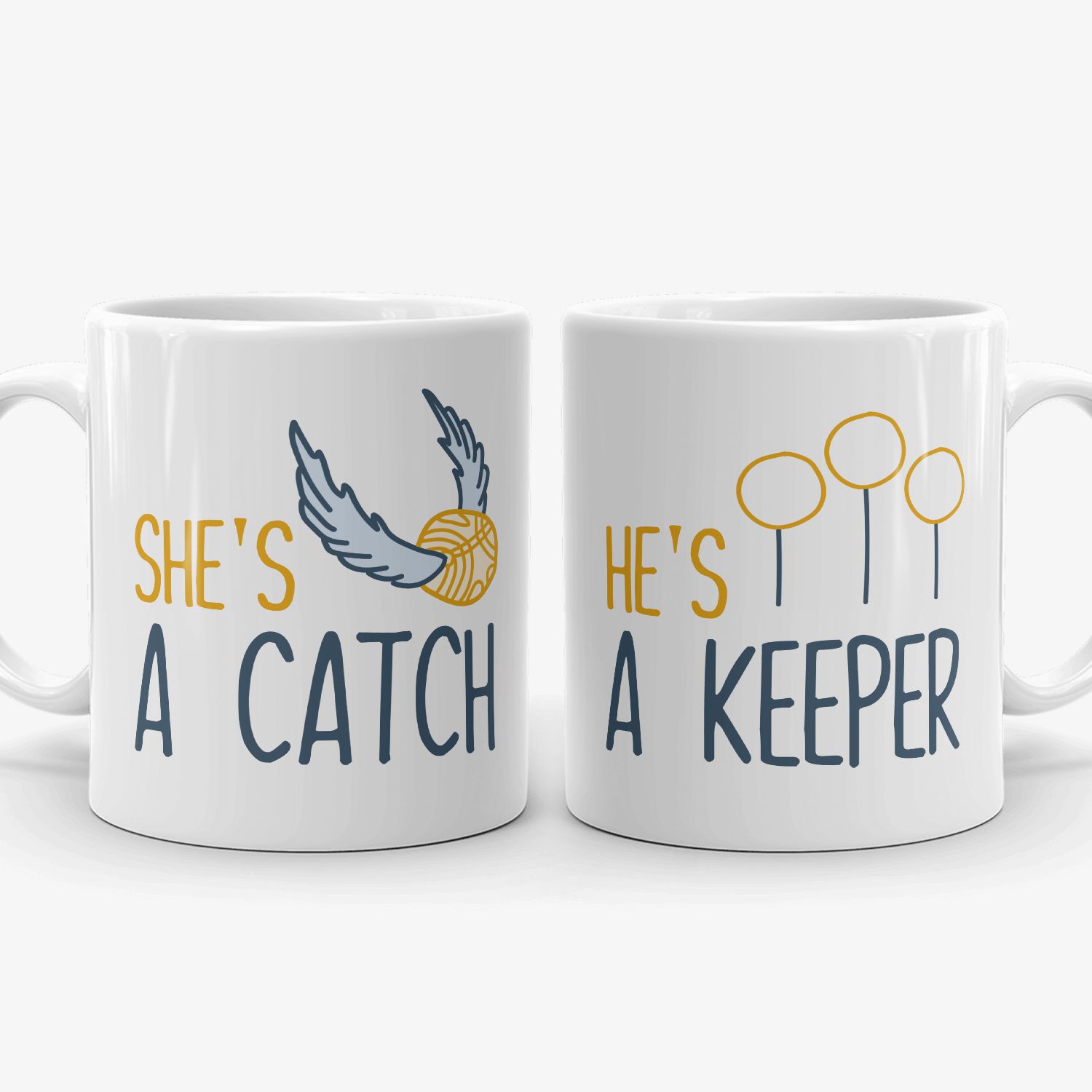This is an image featuring a pair of white coffee mugs specifically designed for Harry Potter fans, particularly catering to a heterosexual couple based on the messaging. The left-hand mug displays the phrase "She's a catch" with "She’s" in a golden color and "a catch" in dark blue. Next to the text, there's a detailed illustration of the iconic golden snitch, with a gold ball and blue wings. The right-hand mug bears the phrase "He's a keeper," where "He’s" is also in gold, and "a keeper" is in dark blue, referencing the Quidditch position. Beside this text, the design features three rings of varying heights, representing Quidditch goals. Both mugs have handles facing outward, and the elegant designs incorporate both text and imagery, making for a charming product demonstration photo.